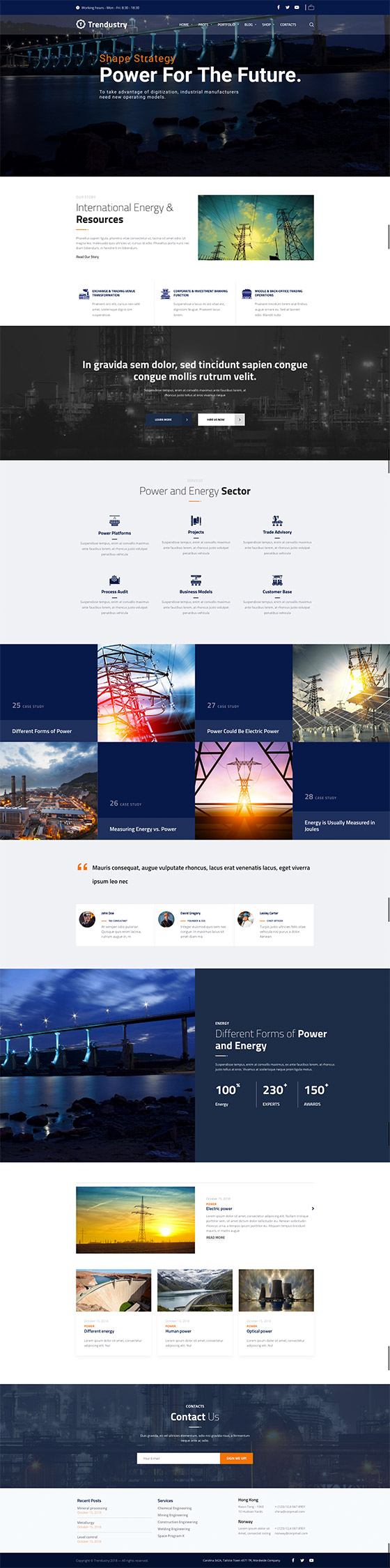A densely packed, tall web page is displayed in a constricted viewing area, making it challenging to read the text clearly. At the top of the page, the headline "Power for the Future" is prominently visible. The content seems related to the power and energy sector, with numerous images of pylons and transmission towers scattered throughout the page, suggesting that it may belong to an electric company or a consultant for such enterprises. The text includes frequent mentions of "power," "energy," and "international energy and resources," interspersed with marketing buzzwords and promotional banners. The overall background color of the webpage is a light shade, either white or light gray, which contrasts with the vibrant banner images. One notably elongated banner features statistical figures like "100," "230," and "150," though the context for these numbers is unclear—they could represent measurements such as feet. Additionally, there is a structure resembling a bridge, potentially used for supporting power transmission cables.